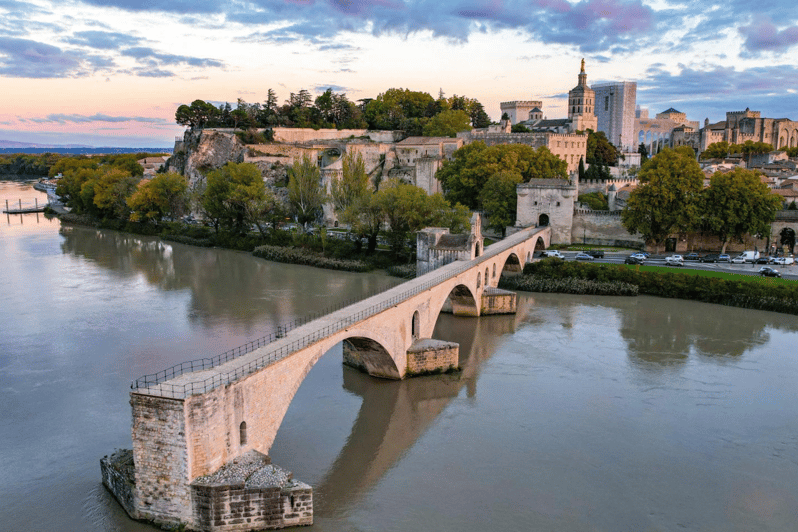The image captures a stonework marvel, possibly the Pont Saint-Benezette, a historic bridge extending partially into the murky brown waters of a river or large lake in France, likely in the evening. The ancient bridge, adorned with black railings on either side, features several arches enabling boats to pass through. Though it appears the structure was constructed to span the water, it terminates midway, resembling a long pier. The bridge originates from a scenic riverbank, lined with trees and a street where cars are seen driving. Among the waterfront, a mixture of old and new buildings can be observed, with a prominent stone building seamlessly connected to the bridge, housing a black doorway. The backdrop of the scene includes an array of tall buildings and an overcast sky, indicating an impending sunset. The tranquil ambiance is enhanced by the surrounding verdant trees and the absence of boats in the water. The detailed perspective, possibly taken from a drone or airplane, offers an expansive view, encapsulating the historic charm and tranquil beauty of the bridge and its surroundings.